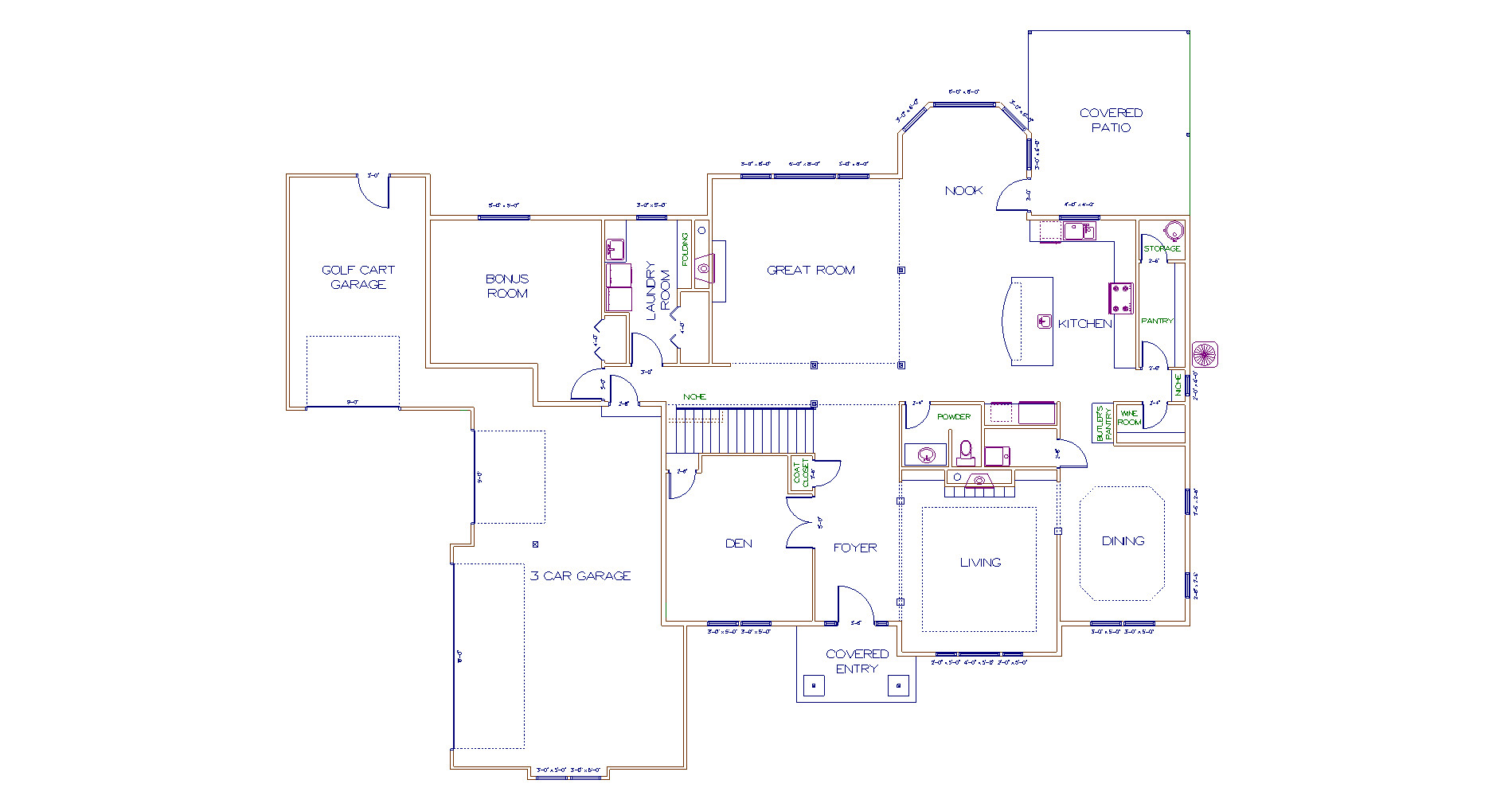This meticulously crafted floor plan, likely designed by a professional draftsman, offers a comprehensive view of a home's layout. The detailed blueprint showcases numerous rooms, including a covered patio, kitchen, dining room, living room, nook, great room, den, foyer, covered entry, three-car garage, laundry room, bonus room, and even a specialized golf cart garage. The schematic, devoid of furniture, provides a clear top-down view as though the roof has been removed. 

Stairs are illustrated with narrow, densely spaced vertical lines, while windows stand out in thick blue lines, and doors are denoted with curved lines. Blue numerical measurements accompany most rooms, highlighting precise dimensions. The drawing features ample white space, ensuring the layout remains uncluttered and easy to read.